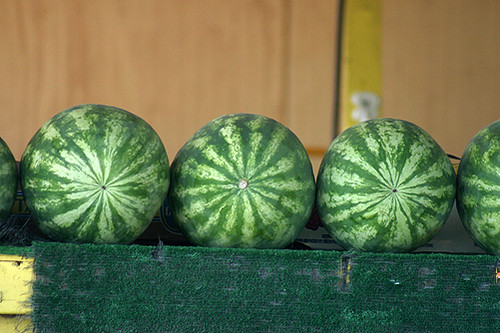This detailed image showcases five similar watermelons, arranged horizontally in a diagonal pattern. They rest on a rough, wooden shelf painted yellow and covered by a coarse green cloth that resembles felt. The shelf itself sits against a light wood panel background with a vertical yellow stripe on the right. Of the five watermelons, three are visible in full from their stem ends, while the fourth is partially visible on the left and the fifth is cut off on the right. The watermelons are pale green with dark green stripes and are positioned so that we see the circular stem areas. The image offers an intriguing perspective, making it unclear if the watermelons are truly diagonal or if the photo was taken at an angle.